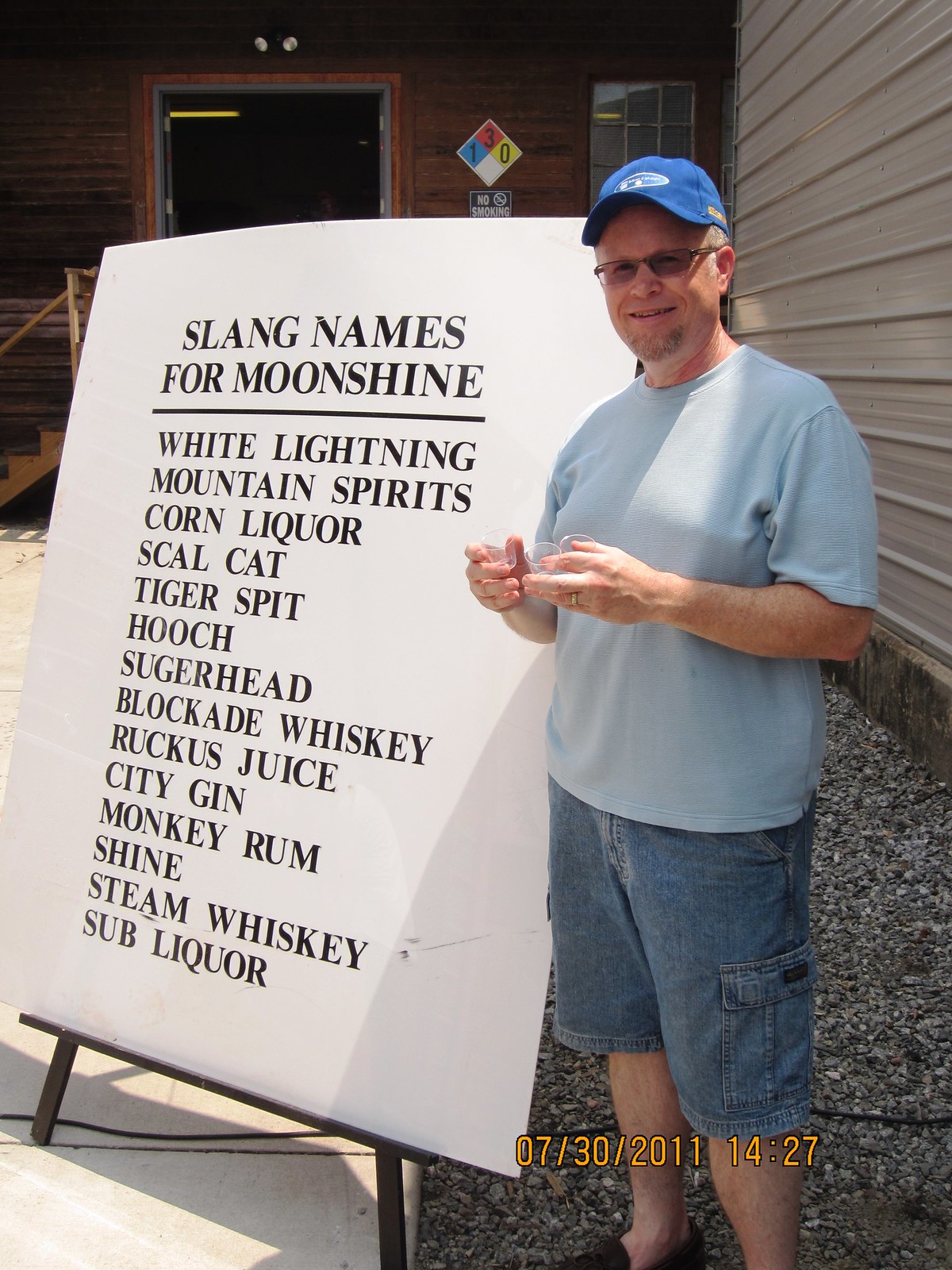In this photograph, a man is standing on a gravelly ground next to a prominent white sign with black handwritten text that lists slang names for moonshine, including “white lightning,” “mountain spirits,” “corn liquor,” “scowl cat,” “tiger spit,” “hooch,” “sugar head,” “blockade whiskey,” “ruckus juice,” “city gin,” “monkey rum,” “shine,” “steam whiskey,” and “sub liquor.” The sign, which is propped up on an easel, has an orange date stamp at the bottom right reading "07-30-2011-1427." The man, who is smiling and wearing a blue baseball cap, sunglasses, a light blue t-shirt, and denim shorts that reach his knees, stands in front of a brown building made of rocks. The building features a large doorway and various signs, including a blue square with a white "1," a red square with a white "3," a yellow square with a white "0," and a no smoking sign. The scene captures a rustic, outdoors setting detailed with a gravelly ground.